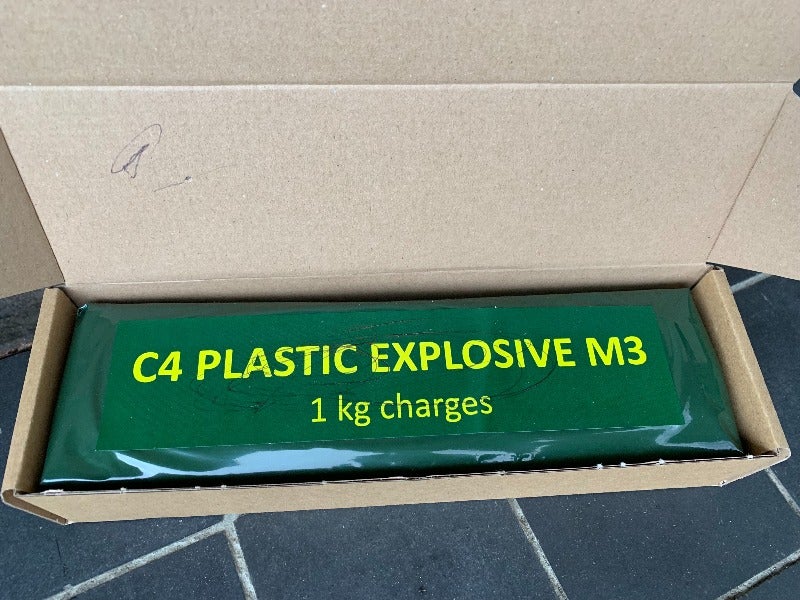This photograph captures a light brown, rectangular cardboard box with its lid open, revealing its contents. The box is set on a floor composed of large, dark grey square tiles with white grout lines. Inside the cardboard box is a dark green plastic container with text in bold, yellow all-capital letters. The top line of the text reads "C4 Plastic Explosive M3," and just below that, "1 KG CHARGES." The detailed placement and visibility of the green container contrasts with the box's mundane appearance, emphasizing the significance of its contents within the simple setting.